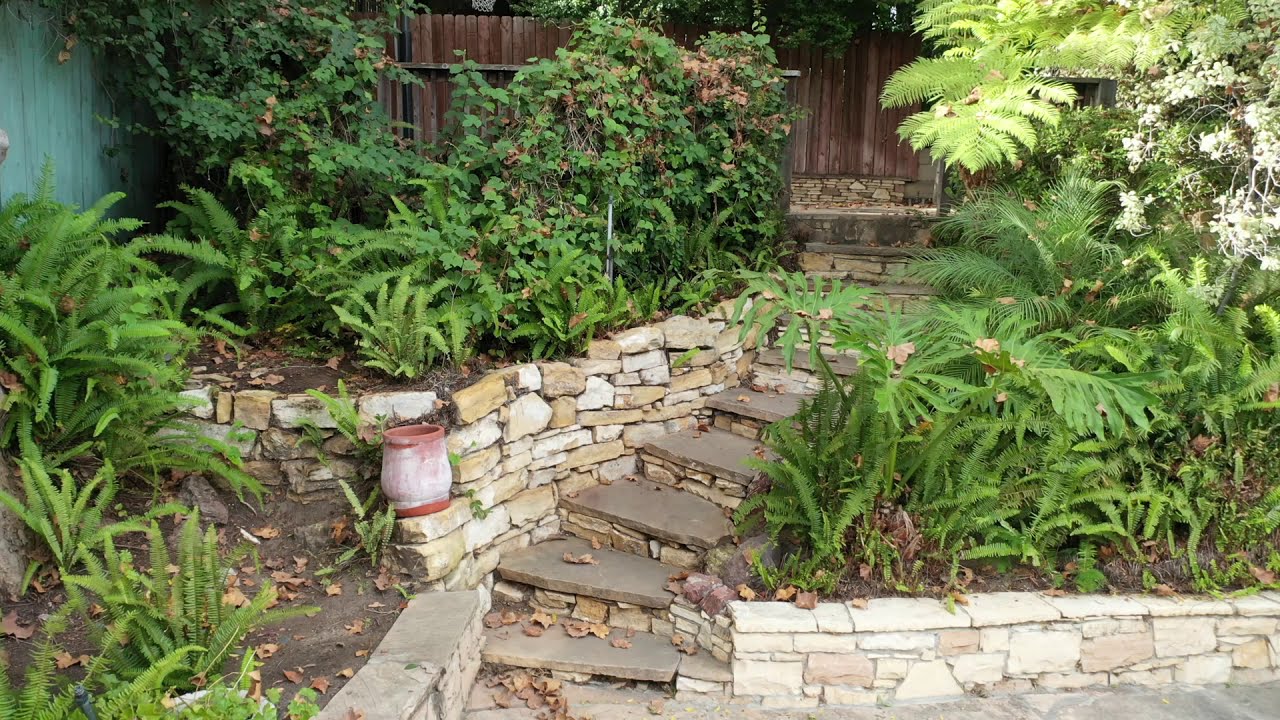The image depicts the stone stairway and garden area of a residence, surrounded by abundant greenery and various types of fern plants. The narrow stairway consists of about six steps, made from beige and brown stone blocks with darker brown treads. The steps curve slightly towards the right as you ascend and are flanked by small retaining walls constructed from individual stones. On the left side, these walls support the lush garden, while on the right side, they hold back dirt from spilling onto the path, which is lined with additional fern plants.

Lying on the pathway is a reddish-brown terracotta pot. The stairway leads up to a brown wooden fence, with an open door that reveals another pathway paved with similar beige and brown tiles. Leaves are scattered across the ground, adding to the natural, slightly untamed aesthetic of the scene, and the overall setting evokes a tranquil, outdoor space richly intertwined with nature.